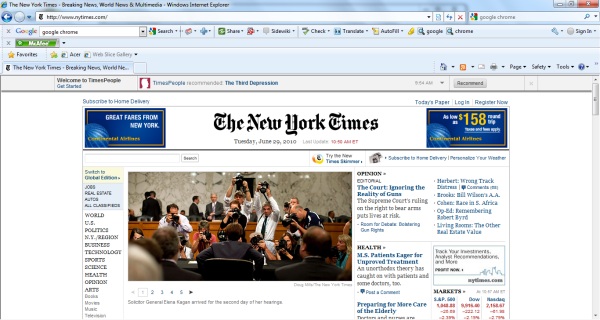A small screenshot captures a light blue-themed Internet Explorer browser window open to the New York Times website. In the top left corner, the iconic Internet Explorer logo is visible. Adjacent to the logo, the browser tab displays the text, "The New York Times - Breaking News, World News, and Multimedia," followed by "Windows Internet Explorer." On the far right, standard window control buttons for minimize and close (X) are present. Below this, an address bar is centrally located, flanked on the right by a search bar.

Beneath the primary navigation, two active extensions are shown. The first extension is from Google, featuring options for search, share, translate, autofill, and links to Google and Chrome. The second extension, from McAfee, is highlighted in green and includes a drop-down box.

Dominating the main view of the browser is the New York Times homepage, which displays a white background with the current front-page content of the news site.